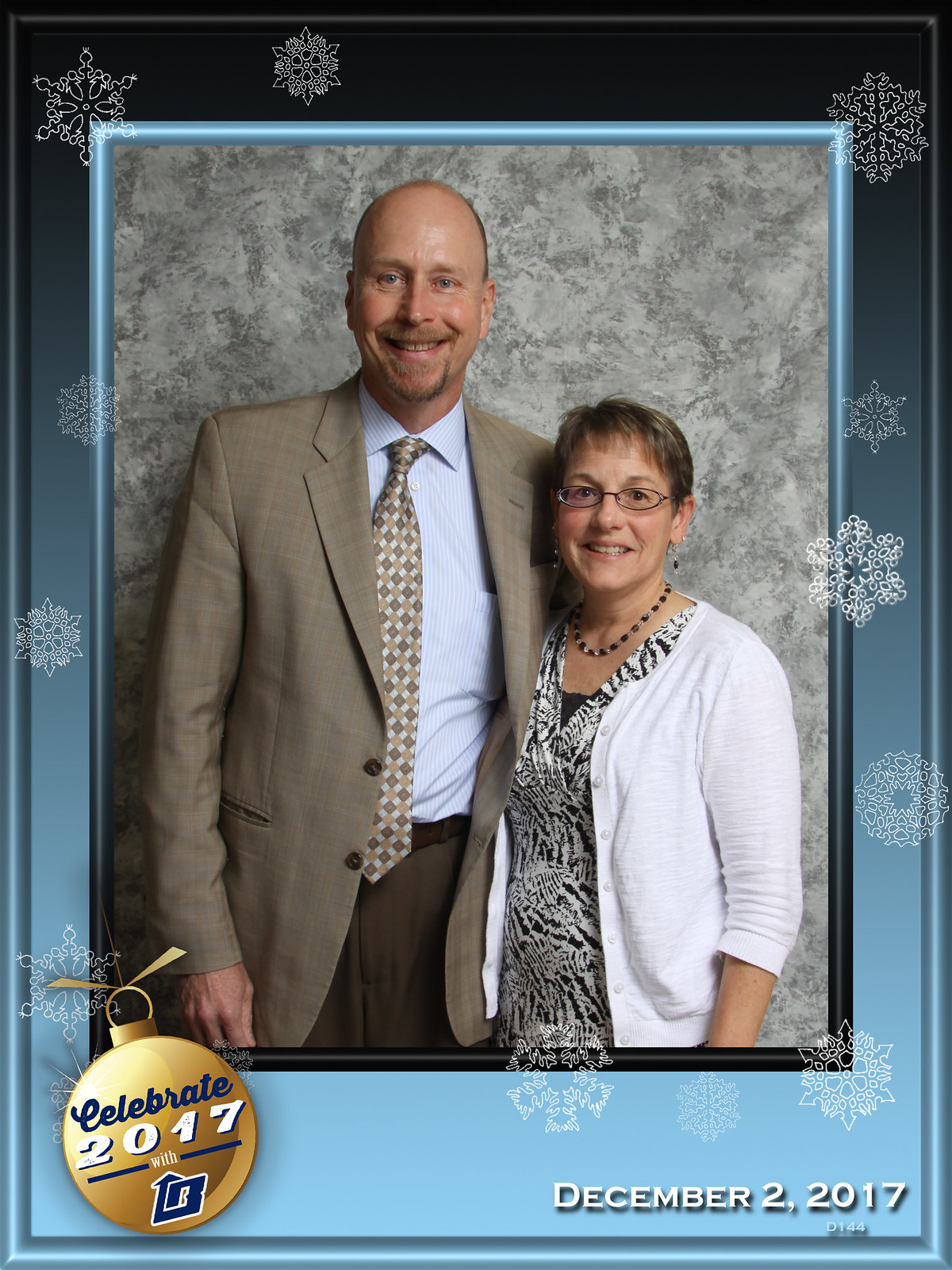The image depicts a family portrait featuring a man and a woman, possibly husband and wife, dressed in semi-formal attire. The man, standing on the left, wears a tan jacket, a checkered tan tie, a blue and white pinstripe shirt, and brown pants. He sports a goatee and is partially bald. The woman, who is noticeably shorter, stands next to him wearing a white jacket over a black and white zebra-print dress. She accessorizes with a necklace, earrings, and glasses, and has short brown hair.

The background of the photo appears to be a marble wall, giving a slightly formal touch to the scene. This portrait is digitally framed within a three-tiered border. The innermost border features a gradient blue hue with falling snowflakes, providing a festive, wintery feel. Surrounding this is a second layer of a silver-gray border that attempts to give a three-dimensional appearance, albeit somewhat cheaply executed. The outermost border mirrors the first in its blue gradient and snowflake pattern.

In the bottom right corner of the image, an ornament shaped like a snow globe reads "Celebrate 2017," with the letters "LB" appearing stylized within it. The date "December 2nd, 2017" is also inscribed there, indicating the time the photo was taken or sent out as a possible holiday greeting. Despite the various design elements and borders trying to enhance its look, the overall impression remains modest.